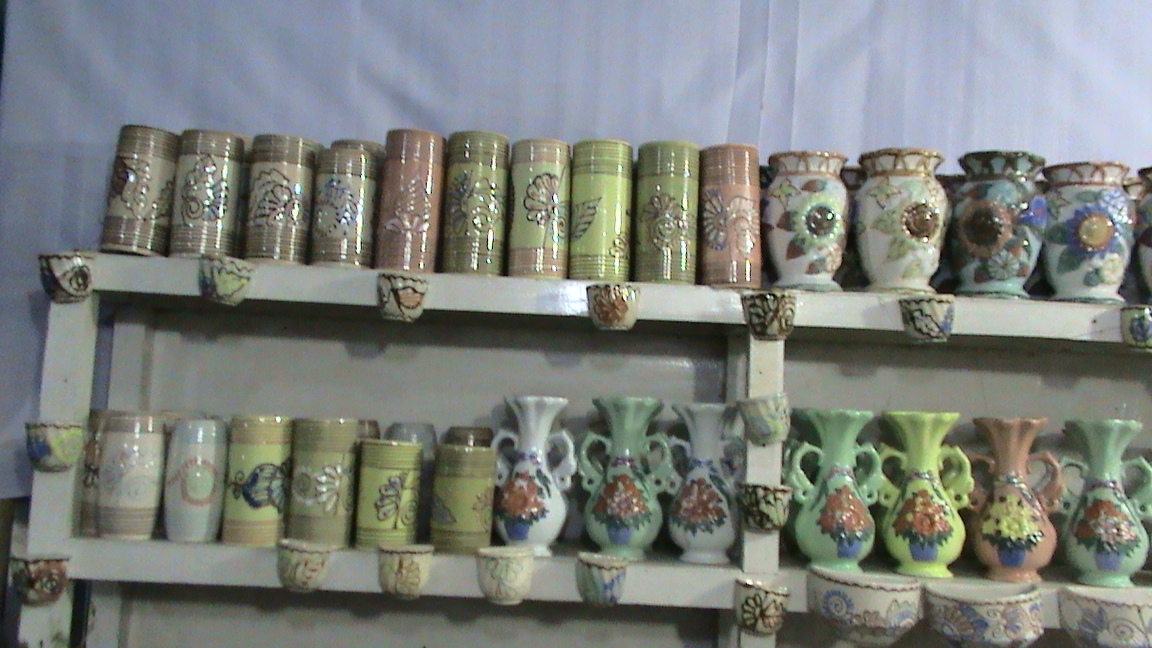The image captures a detailed arrangement of variously colored and styled ceramic vases and cups, aligned meticulously on the top two shelves of what appears to be a bookshelf or potter's shelf. The background behind the shelves is a light gray or off-white fabric, enhancing the display's aesthetic. 

On the top shelf, starting from the left, there are four ceramic pieces shaped like beer cans, featuring intricate designs resembling seashells. These are followed by six taller, thinner vases, and then a typical shorter, wider vase with the top half flaring outward. The vases on this shelf are primarily in shades of green, pink, teal, and white, with some showcasing floral patterns.

The second shelf showcases six shorter, pastel-colored, beer-can-shaped vases aligned to the left. To the right of these, there are seven traditional-style vases with larger bases, elongated necks, and flared tops, each adorned with two small handles. The colors prominently include greens, yellows, pinks, and the occasional light blue, further embellished with floral designs, reinforcing the impression that these are indeed designed as flower vases.